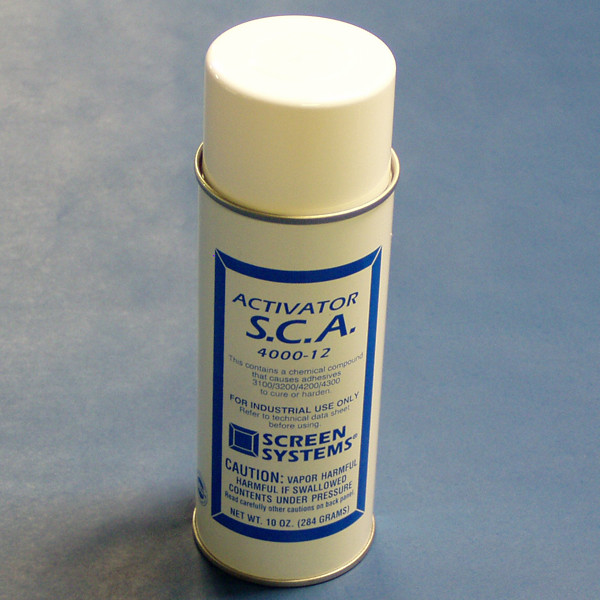This image displays a close-up shot of a white aerosol canister situated against a sky blue background. The canister is centered in the image. It has a white cap and features metal rims encircling the top and bottom. In the middle of the can, there is a blue label. Prominently printed at the top of the label are the words "Activator SCA" followed by the number "4000-12." Below this, text indicates that the can contains a chemical compound designed for adhesives, leading to curing or hardening. Additional warnings and instructions are present on the label, including "For industrial use only," "Refer to technical data sheet before using," "Caution: Vapor harmful," "Harmful if swallowed," and "Contents under pressure." The label also advises reading additional cautions on the back panel. The net weight of the canister is noted to be 10 ounces (284 grams). The logo and the phrase "Screen Systems" appear in blue bold text on the label. The detailed and numerous cautionary messages emphasize the industrial and potentially hazardous nature of the product.